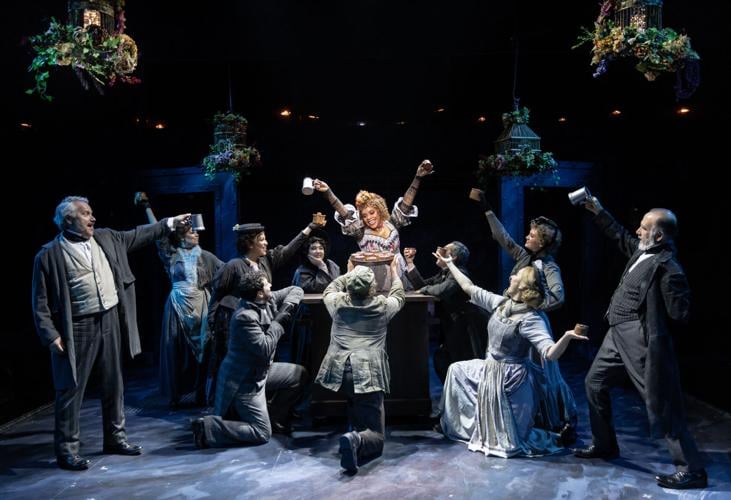In this evocative stage play scene, a jubilant group of people is captured mid-toast, celebrating one central figure amongst them. The men are garbed in dark jackets and trousers, reminiscent of period costumes, while the women don flowing, light-colored dresses, adding an ethereal quality to the tableau. Center stage, a triumphant woman strikes a victory pose, her fists raised high, clutching a light-colored mug indicative of a celebratory drink. Bracketing the composition, two men also hold similar light-colored cups, enhancing the festive atmosphere.

Kneeling before a small box, several individuals extend their hands toward the woman in the background, emphasizing her central role in the scene. A man, prominently positioned in front of the box, supports a tray laden with what appears to be an assortment of treats or food, suggesting communal sharing and revelry. 

Behind this animated assembly, the backdrop features a delicate, light-colored garden archway or pathway, adorned with floral designs that crown its apex. The dark stage floor contrasts sharply with the ensemble's attire, while dim yellow and white spotlights cast a subtle glow from above, illuminating the scene and highlighting the dramatic ambiance of the play.